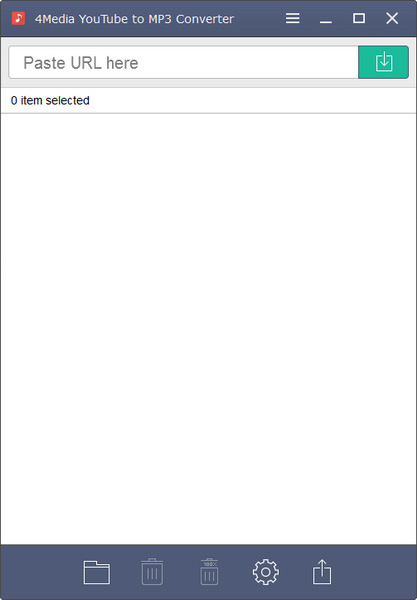The screenshot depicts the interface of a "YouTube to MP3 Converter" application. The top bar of the application shows the typical window control buttons: Minimize, Maximize, and Exit. There is a clearly displayed text box labeled "Paste URL here," positioned above a prominent green "Download" button. The interface currently indicates that there are zero items selected. The main area of the application is a white screen, likely intended for displaying download progress or selected items. At the bottom of the interface, there are several functional icons including a folder, two trash cans, settings, and an upload button. This layout aims to simplify the user experience for converting and managing YouTube videos to MP3 files.